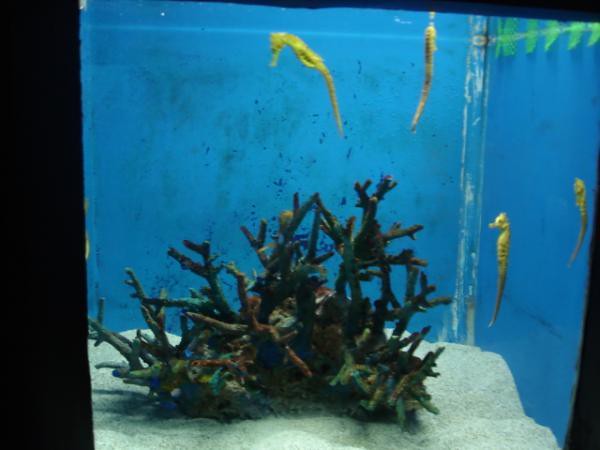The image is a low-quality, square aspect ratio photograph, likely taken with an old digital camera, capturing a small aquarium with a solid blue background. The aquarium is viewed from the front, the only visible glass part, with black shadows surrounding it, offering no hints about its surroundings. Inside, the aquarium features clean, white sandy bottom and a prominent, large coral-like structure in the center, reaching almost the entire width and about half the height of the tank. This coral structure exhibits shades of blue with some copper-tinted areas, adding to its vivid appearance. There are four small, thin yellow seahorses, presumably juveniles, positioned at various points within the tank: two seahorses float near the water’s surface, one seahorse is positioned to the left with its face down and tail hanging, and the last seahorse is near the bottom right corner, facing left. The aquarium is illuminated by a light source from above, casting a gentle glow on the scene.